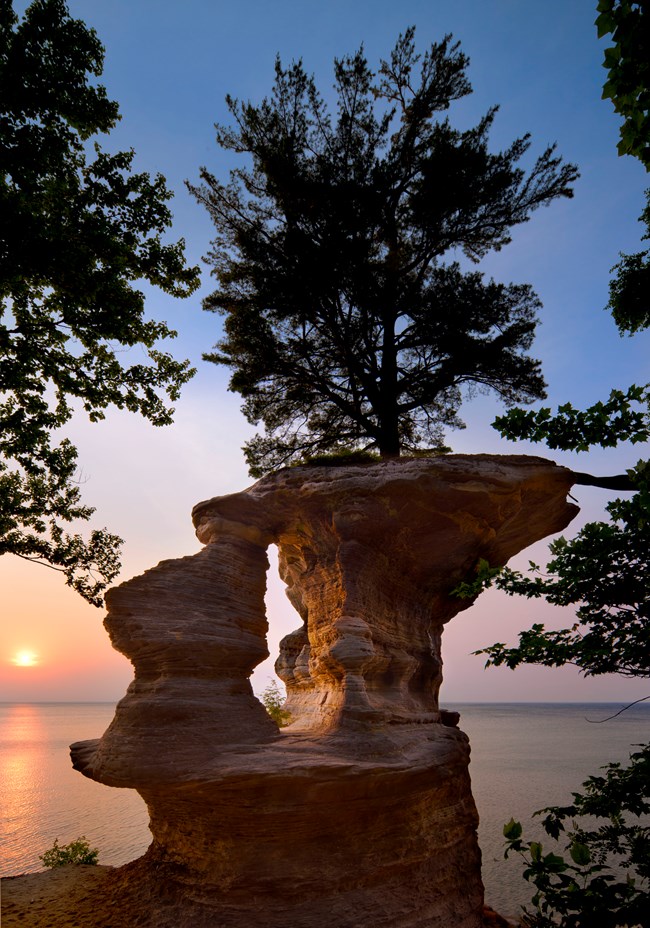The image captures a serene, picturesque scene at the shore near a large body of water, potentially a lake or ocean. At its center stands a striking sandstone rock formation, sculpted by long-term erosion into a unique, tower-like structure with a small pine tree perched gracefully at its top. This light brown, sandy-colored formation is flanked by additional trees on both the left and right sides of the image, adding depth and natural beauty. In the foreground, patches of sand suggest a gentle, coastal environment. The expansive, calm water stretches to the horizon in the background, reflecting the warm hues of the setting or rising sun. The sky transitions from a deep blue at the top to vibrant shades of pink, orange, and red closer to the horizon, enhancing the tranquil and majestic atmosphere. A soft reflection of the sun's light shimmers on the water, blending harmoniously with the pristine blue, creating a captivating visual symphony of nature's elements.